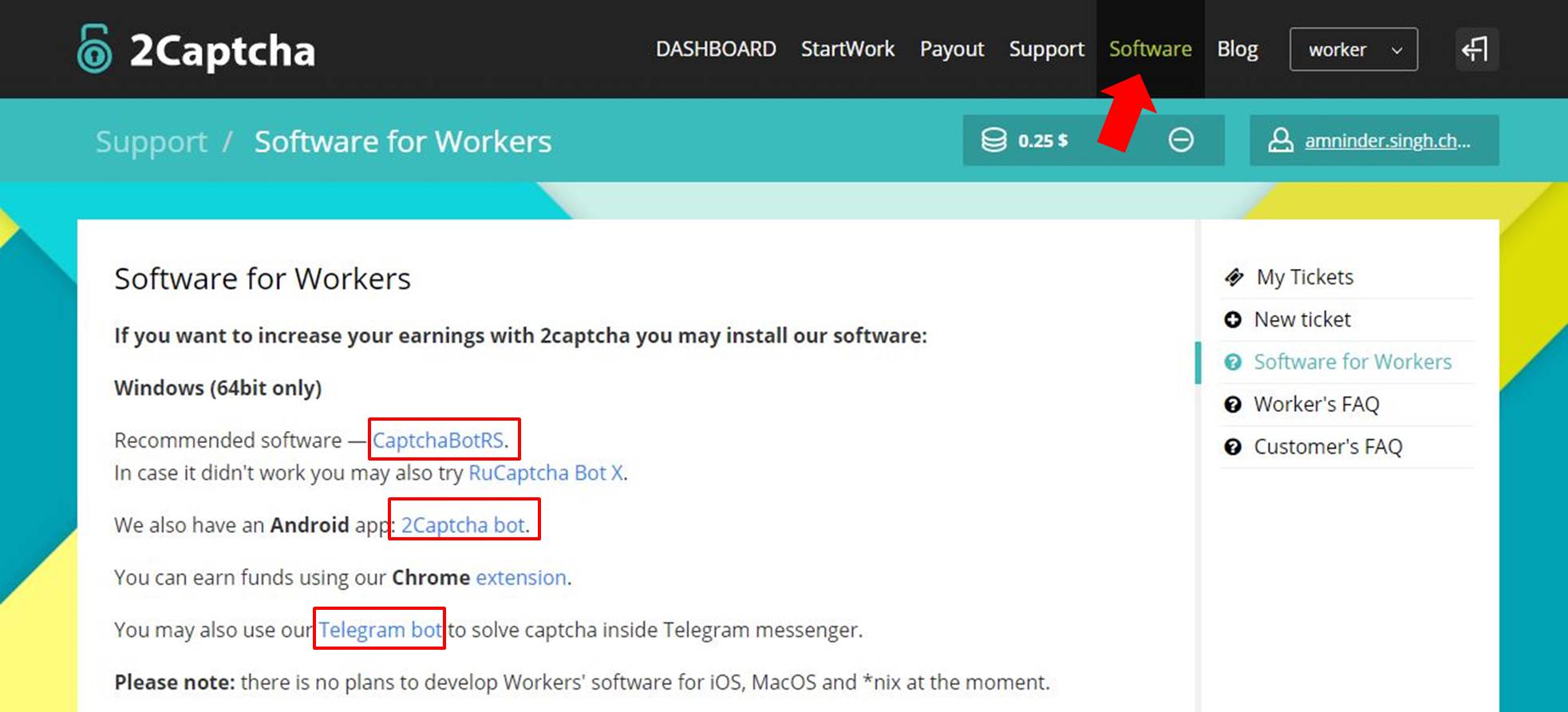This image is a partial screenshot of a webpage from the site "2CAPTCHA." The bottom section of the webpage is missing, making the image incomplete. The webpage features a logo with a blue lock icon at the top, accompanied by a black banner that includes navigational links labeled "Dashboard," "Start Work," "Payout," "Support," "Software," and "Blog." There is also a visible drop-down menu for additional options.

A large red arrow points to the "Software" tab, indicating that the user is currently on the software page. The main content area of the page features a blue and yellow color scheme with geometric shapes in different hues of blue and yellow. Dominating the center of the page is a prominent white box containing text that addresses workers: "Software for workers. If you want to increase your earnings with 2CAPTCHA, you may install our software, Windows 64-bit only." Below this message are download links for the software program, tailored to Windows 64-bit systems.